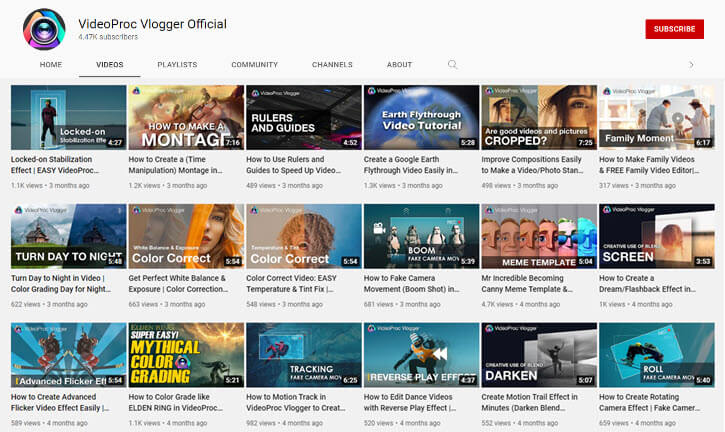The image is a screenshot from the VideoProc Vlogger official website. Prominently displayed at the upper center is the website's logo, featuring an icon resembling a camera lens surrounded by a spectrum of colors, symbolizing video recording. In the top right corner, there is a vibrant red "Subscribe" button.

Directly beneath the logo, a navigational menu bar spans horizontally with sections labeled: Home, Videos, Playlist, Community, Channels, and About. To the far right of this menu sits a grey magnifying glass icon, indicating the search function.

Below this menu, the interface displays clickable sections that provide various information and tutorials. These sections are arranged in three rows, each with six thumbnails, making a total of 18 interactive elements. Among the visible titles of these sections, users can find topics such as "Locked-on Stabilization," "How to Create a Time Manipulation Montage," and a variety of other instructional video topics.